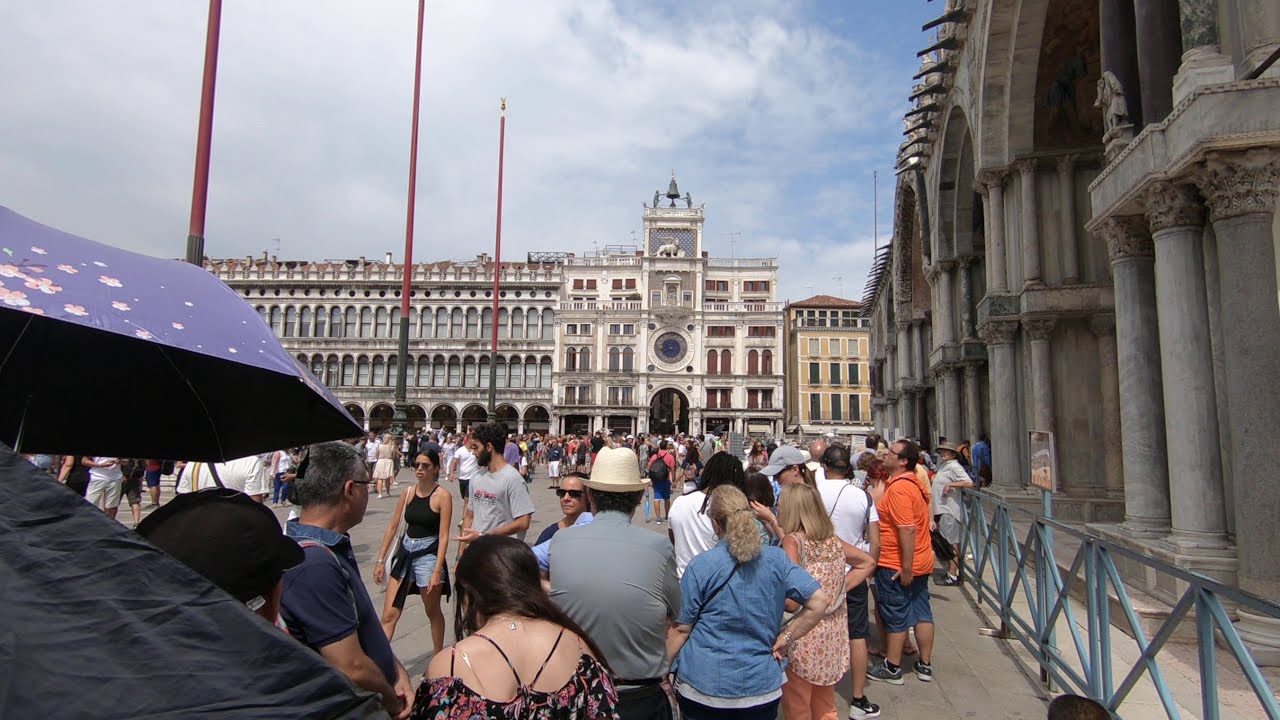The image captures a bustling European town square on a hot summer day. People are out and about in shorts and short-sleeved shirts, indicating the warmth of the day. The crowded street is filled with perhaps over a hundred people, likely a mix of tourists enjoying their vacations and locals conducting daily business. The scene is shot in landscape orientation, with a view slightly from above, possibly from a nearby staircase.

Dominating the background is a tall, approximately five-story European building with numerous rounded windows, indicative of traditional architectural styles. On the right side, there's an older stone building distinguished by its gray color, pillars, and a blue metal fence. Amid the crowd in the lower left corner, a vibrant purple umbrella dotted with pink flowers stands out. Three tall poles with red tops reach into the partially clouded sky, which occupies the upper left and middle parts of the image. A silver guardrail with X-shaped patterns can be seen in the bottom right corner. Overall, the image effectively captures the lively atmosphere and architectural charm of this European urban setting.